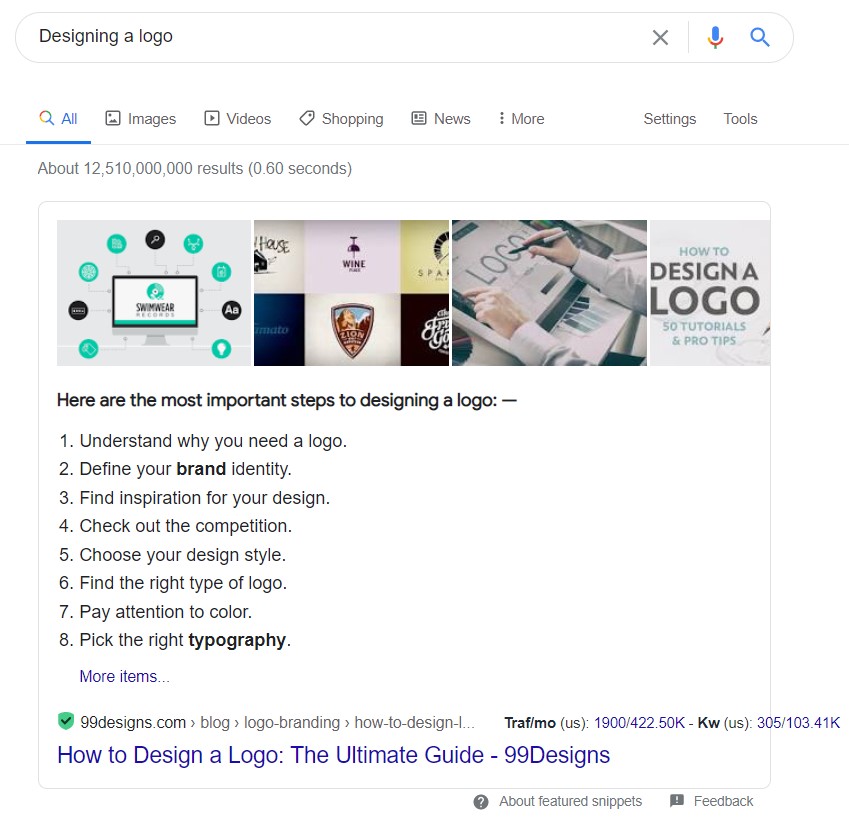This image captures a Google search results page for the query "designing a logo". At the top of the image, the search bar extends horizontally across the screen, but the "Google" logo is not visible. The query "designing a logo" is prominently displayed within the search bar.

Below the search bar is a navigation menu containing several tabs: "All," "Images," "Videos," "Shopping," "News," and "More." Adjacent to these tabs are the "Settings" and "Tools" options. The search results indicate approximately 12,510,000,000 results.

The first search result is from 99designs.com and includes four thumbnail images at the top. Beneath these thumbnails is a list titled "Here are the most important steps to designing a logo." The first item on this list is "Understand why you need a logo."